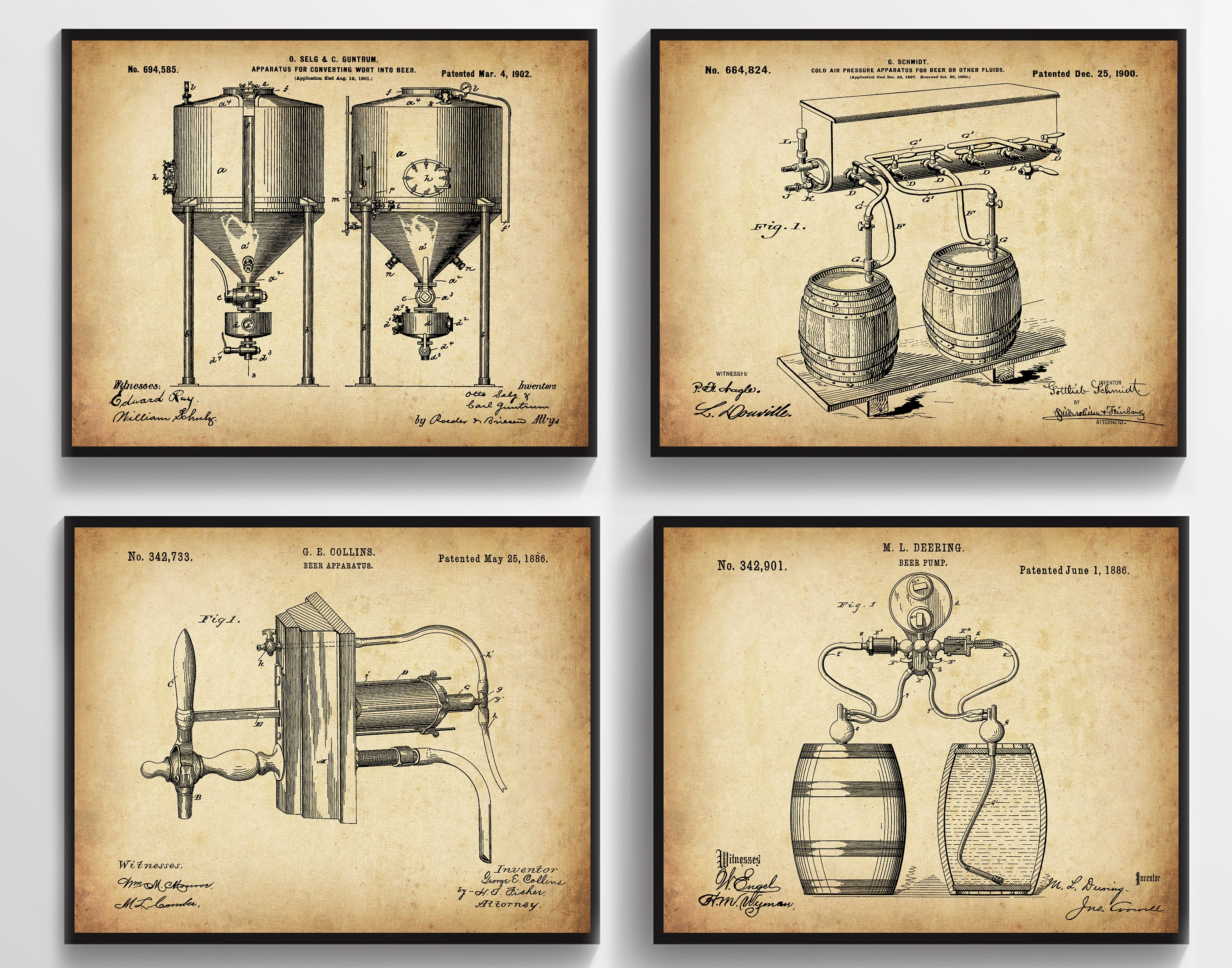The display features a set of four framed illustrations, each enclosed in a thin black frame, uniformly hung on a light grey wall. The illustrations, printed on aged beige paper that gives an antique appearance, depict various apparatuses related to beer production. The top left image is labeled "Apparatus for Converting Wort into Beer" and shows detailed drawings of tanks and containers with funnels, tubes, and hoses, resembling water towers. The top right illustration, titled "Schmitt's Cold Air Pressure Apparatus for Beer or Other Fluids," features a sophisticated diagram of tanks connected to barrels via a series of hoses. The bottom left illustration, marked with the date "Patented May 25th, 1886," presents a beer dispensing tap. Lastly, the bottom right image, labeled "M.L. Deering Beer Pump," depicts a mechanical pump connected to two barrels, complete with hoses and nozzles. These vintage diagrams offer a fascinating glimpse into historical beer production equipment.